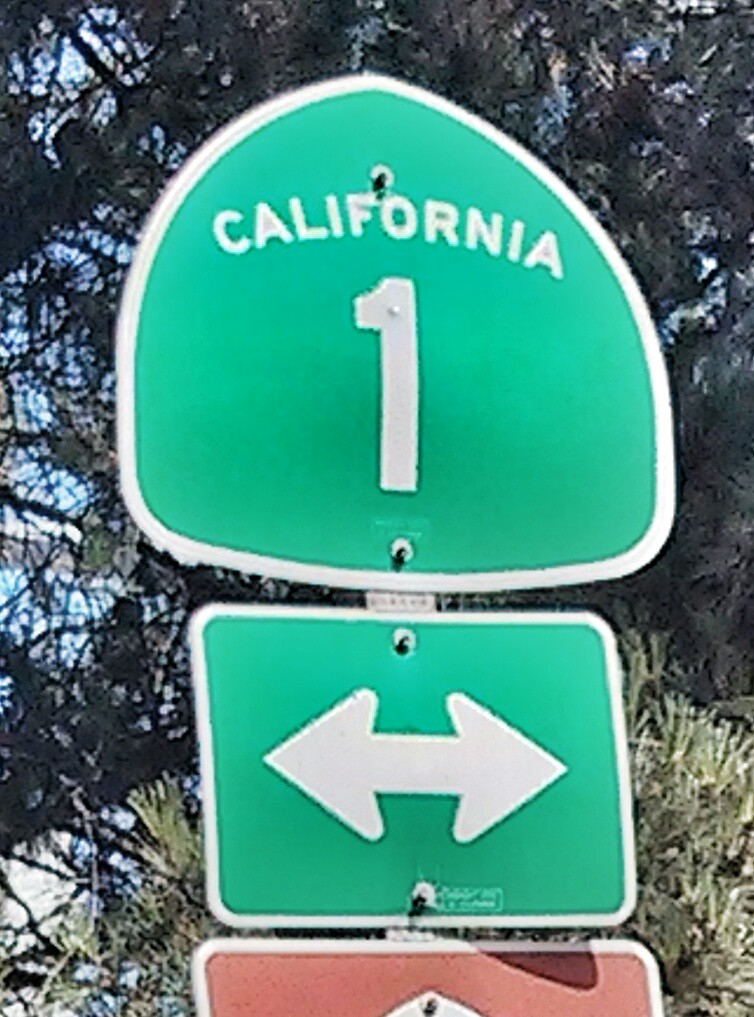The image features a distinctive California Route 1 street sign mounted on a silver pole. The upper sign is green and shaped like a rounded triangle, reminiscent of an inverted teardrop with a point at the bottom. It is securely fastened to the pole with visible bolts. Below it is a green, square sign that harmonizes in color, displaying directional arrows pointing both left and right. Additionally, there is a partial view of a red sign at the base, obscured except for a small white speck, making its exact message unclear. The background reveals two trees: a taller one with broad leaves and a shorter one characterized by needle-like foliage, creating a natural backdrop for the street signs.